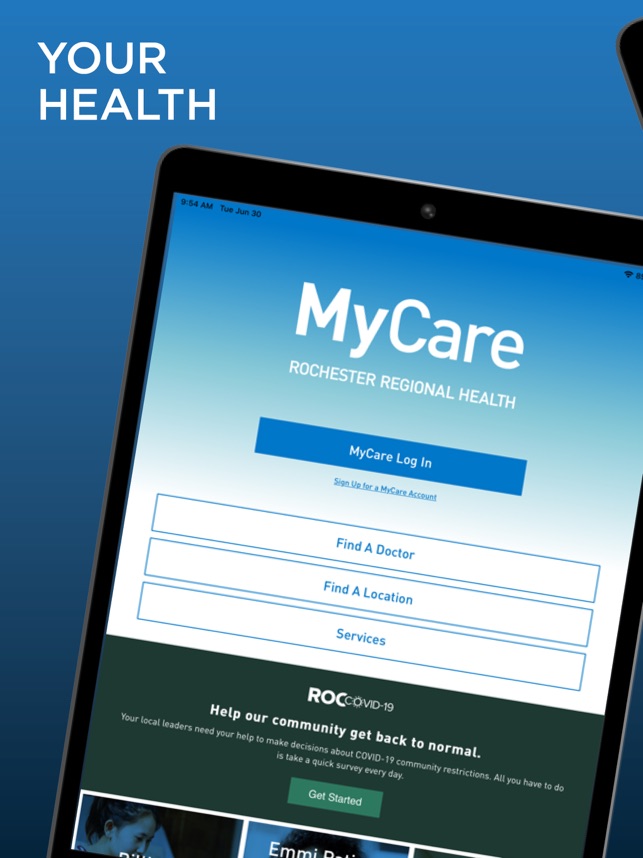This is a screenshot of a landing page for RocHealth. Prominently featured is an image of a cell phone. In the upper left corner, "Your Health" is written in white text on a blue background. On the cell phone screen, there is a blue-to-white gradient with "My Care" displayed in white text in the upper half. Below that, "Rochester Regional Health" is visible along with a blue button labeled "My Care Login." 

Adjacent to the cell phone image, there are three buttons outlined in blue with white backgrounds and blue text that read: "Find a Doctor," "Find a Location," and "Services." 

Beneath these elements, a section with a black background highlights the message, "ROC COVID-19 Help Our Community Get Back to Normal," accompanied by a "Get Started" button. Further down, there appears to be a row of three images. The first image partially shows the top of a person's head, while the remaining visuals are not fully discernible.